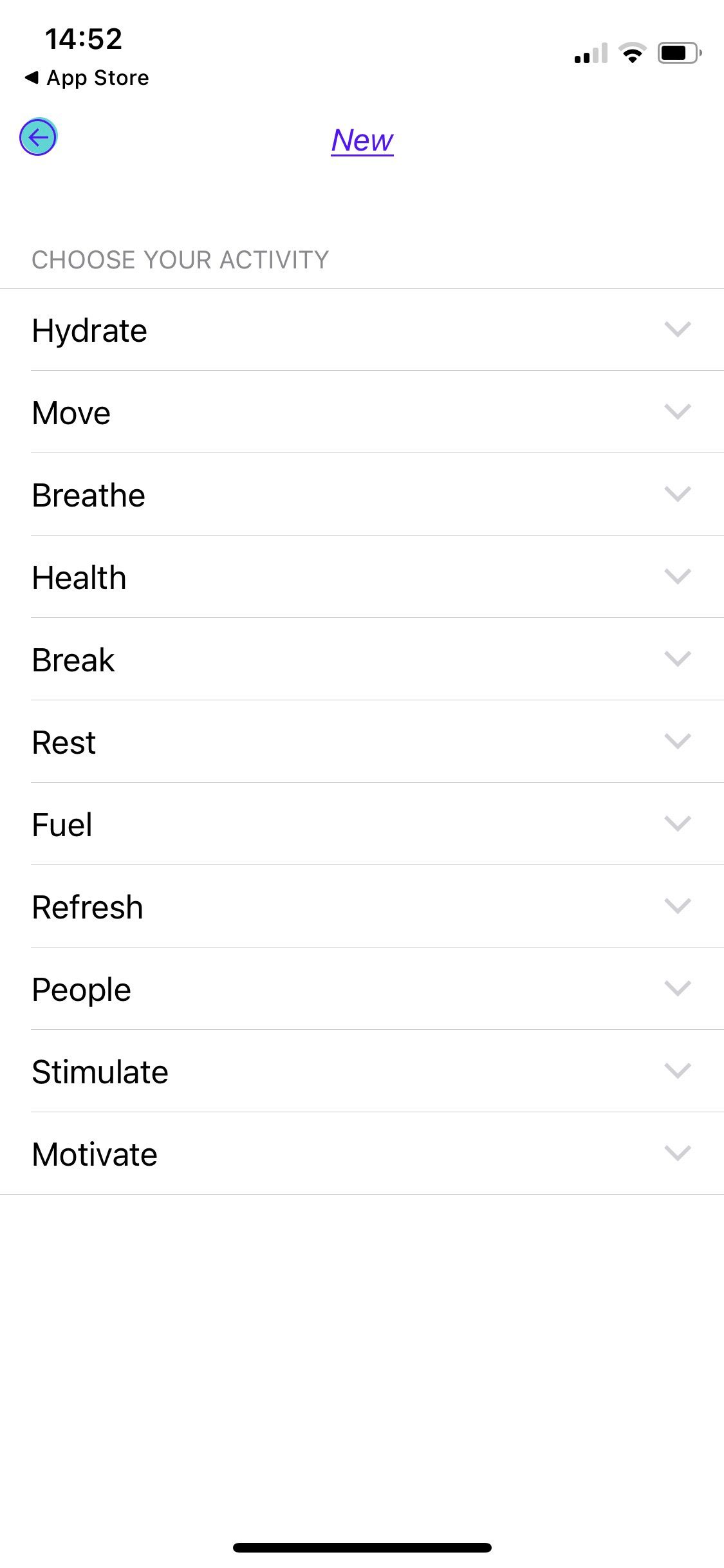Screenshot of an iPhone displaying an app interface. The status bar at the top shows the time as 14:52, 2 out of 4 bars for cell service, 2 out of 3 bars for Wi-Fi, and approximately 60-70% battery life. The interface suggests that the screen was redirected from the App Store, indicated by a back arrow and 'App Store' text on the top left. 

The app features a clean, minimalistic design with black text on a white background and subtle gray lines separating different sections. At the top of the screen is a heading titled "Choose Your Activity." Below this heading is a list of selectable activities, each accompanied by a drop-down menu on the right side. The activities listed from top to bottom are: Hydrate, Move, Breathe, Health, Break, Rest, Feel, Refresh, People, Stimulate, and Motivate. The overall design is simple and user-friendly, focusing on functionality with a straightforward layout.